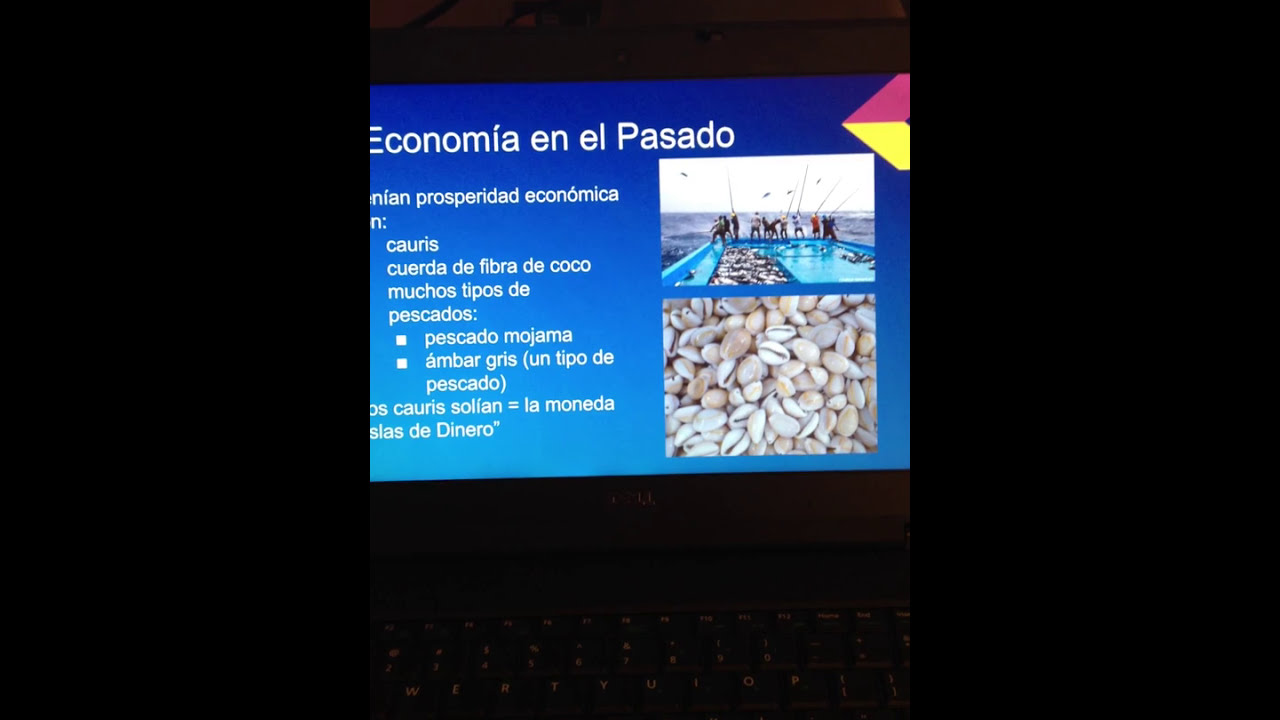In a dimly lit room, a digital photograph captures the screen of an illuminated laptop. The screen displays a webpage or digital pamphlet titled "Economia y El Pasado" in a foreign language. This webpage features a black rectangular background with a prominent blue square on the left side containing white text. To the right of this text, two distinct images are stacked vertically. The top image depicts approximately ten people holding fishing rods, standing on the edge of a large blue boat amidst a rough sea under a white sky. The bottom image showcases an array of white and light brown seashells. The laptop's keyboard, partially visible and gently glowing in the low light, adds depth to the overall composition, with the rest of the surrounding area fading into darkness.